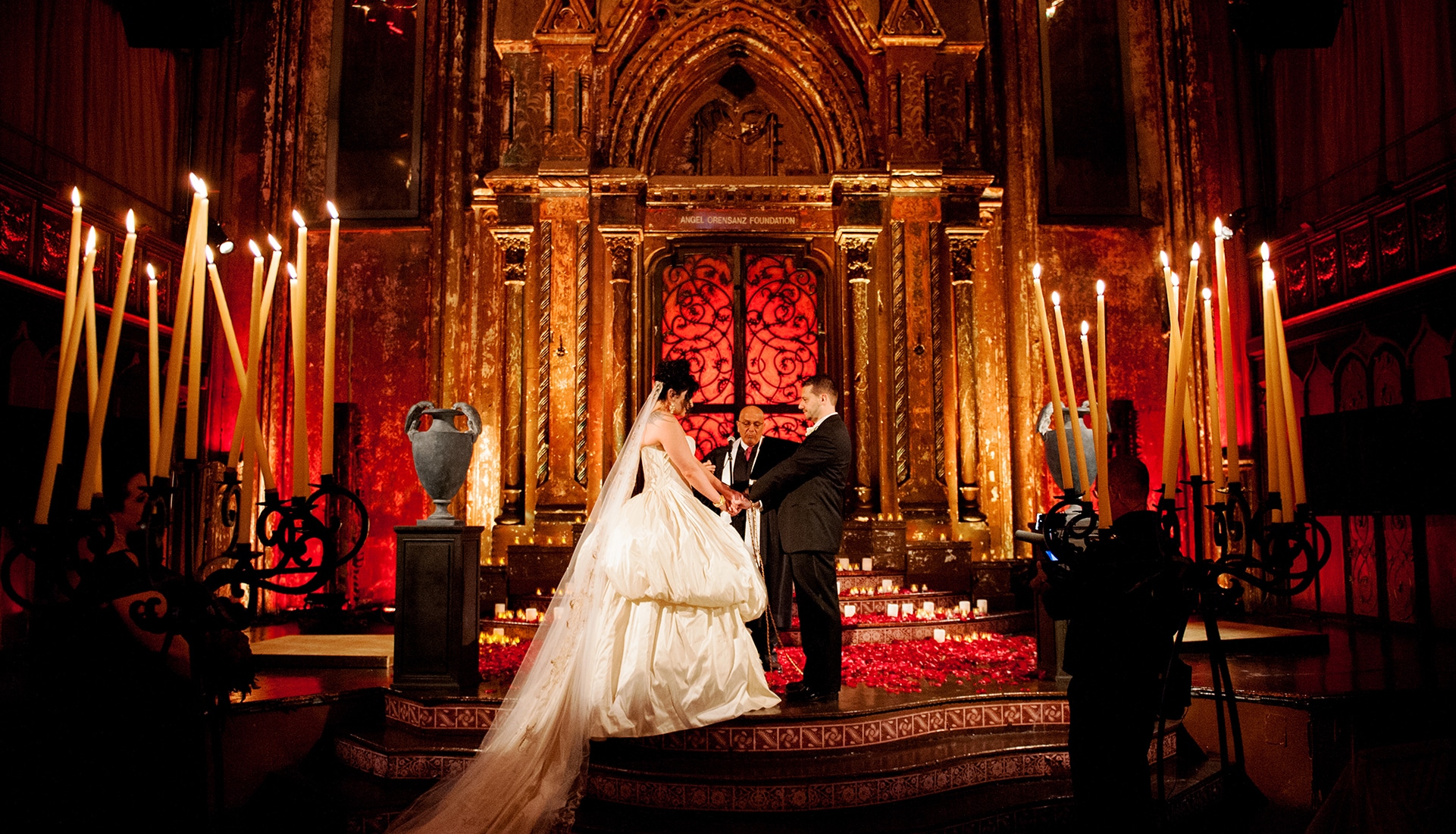The photograph captures a wedding ceremony taking place inside a dimly lit, ornate cathedral. The image, horizontally aligned, features a central aisle that leads to a tastefully decorated altar. The background is adorned with an archway featuring intricate gold and brown stonework, highlighted by illuminated orange tones and red windows, adding an elegant and warm ambiance. 

Tall, elegant candle holders with lit, beige-colored candles, roughly ten to fifteen on each side, frame the scene, casting a soft glow. Standing on two wooden steps with red-tiled risers are the bride and groom. The bride, in a voluminous, poofy white dress with a long, flowing veil, faces the groom, who is dressed in a black suit with a white shirt. They are holding hands in front of the officiant, who is positioned behind them. 

To the side, a photographer captures the moment, his presence subtly highlighted in the composition. Gray pottery and scattered red petals, accompanied by small white candles, add to the decor around the couple, bringing a romantic touch to the altar setting. The overall mood of the photograph is solemn yet celebratory, marked by the intricate details and soft lighting that define the sacred space.